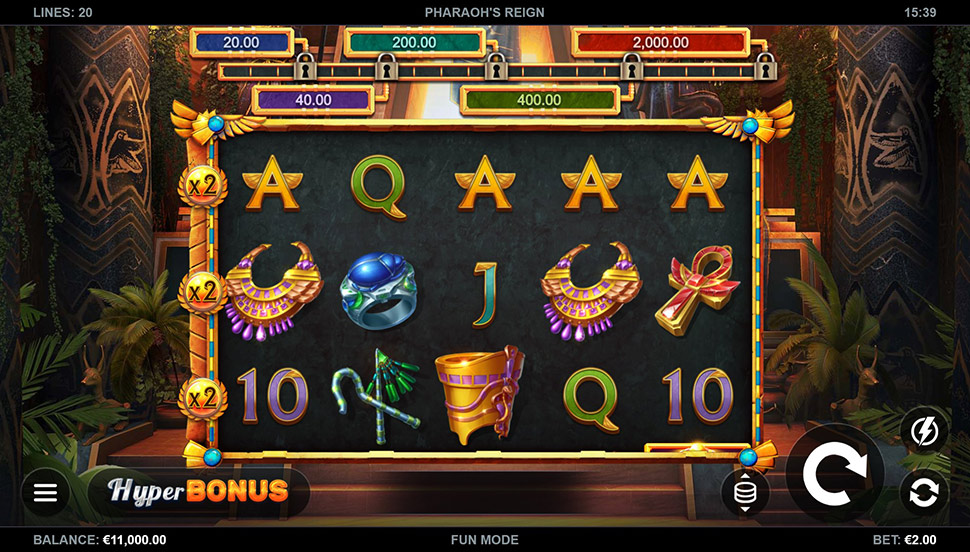The image appears to be a screenshot of an Egyptian-themed online slot machine game titled "Pharaoh's Reign." At the very top of the screen, there is a black bar with white text that reads "LINES: 20" on the left, "Pharaoh's Reign" centered, and "15:39" on the right, possibly indicating the remaining time. Below is a game board filled with various animated symbols indicative of Egyptian culture, such as medallion necklaces, blue rings, flying Ankhs, and letters like A, Q, J, and 10. 

The game board is structured into multiple rows with a 2x multiplier indicated on the left. The top row features symbols like an "A" followed by a "Q" and then three "A"s, alongside a necklace, a blue ring, and a "J." The middle row contains a necklace followed by an Ankh while the bottom row displays a "10," a Staff of Life, a golden bucket, a "Q," and another "10." 

Above the game board, there is a chart of progress in various colors (blue, teal, purple, red, and green) representing different point thresholds (e.g., 20.00, 200.00, 2000.00), but most sections are locked with golden locks and dashes symbolizing progress yet to be made.

At the bottom of the screen, the left black bar indicates a balance of "11,000 euros" and the game is in "FUN MODE." The right side shows the current bet as "2 euros." Below the game board, there are functional buttons including one labeled "HYPER BONUS" in a black rectangle, "BONUS" in orange, and additional buttons for repeat, lightning mode, and coin adjustments on the far right.

In the background, subtle Egyptian architectural elements such as pillar hieroglyphics and statues are partially obscured by leafy patterns, enhancing the thematic experience.